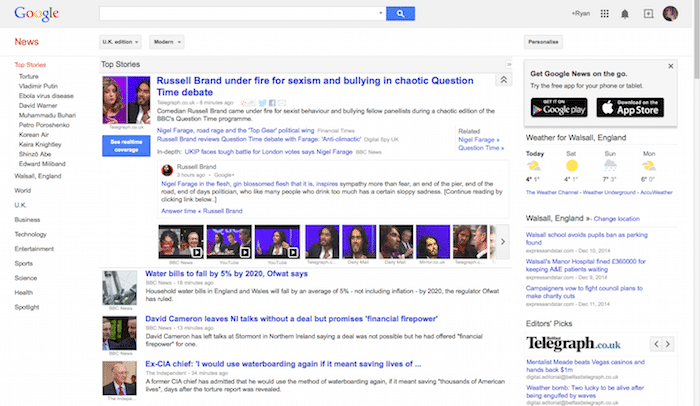An image portrays a screenshot of a Google search results page. The search query itself is not visible within the search bar, but the top two search results are clearly displayed. 

The first search result is a news article titled "Russell Brand under fire for sexism and bullying in chaotic Question Time debate." This suggests that the article discusses allegations against comedian Russell Brand regarding inappropriate behavior during a Question Time debate. The title is highlighted in blue, indicating an active hyperlink.

Beneath this, the second search result is another news article, titled "Water bills to fall by 5% by 2020, Ofwat says." This implies that the regulatory body, Ofwat, has predicted or announced a reduction in water bills by 5% by the year 2020. This title is similarly highlighted in blue, confirming its clickable nature.